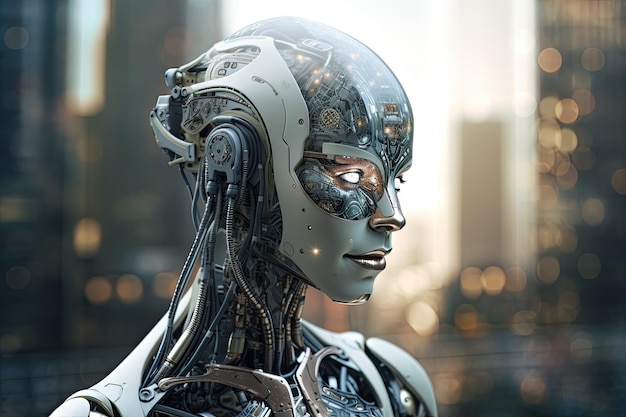This image appears to be a highly detailed, computer-generated photograph set in an outdoor environment. Capturing a side profile, it features a humanoid, possibly feminine robot. The robot's head is turned from left to right, and its face, which resembles that of a woman, lacks hair and is partially transparent. The forehead area is made of glass, revealing intricate circuit boards that make up the "brains." Instead of a human ear, there is a knob with wires extending from it down to the rest of the robot's metallic body.

The shoulders of the robot are semi-transparent, revealing black circuit boards or electronic components underneath. The body itself is primarily metallic, with shades of grey, blue, and some brown. White eyes give the robot a lifelike appearance, although the entire scene remains distinctly mechanical. Some lights blink within the head and body of the robot.

The backdrop features a blurry city skyline that evokes a cyberpunk, futuristic ambiance, complete with tall skyscrapers and illuminated windows. This bustling yet indistinct cityscape enhances the overall sci-fi atmosphere of the image. There is no text accompanying the image.